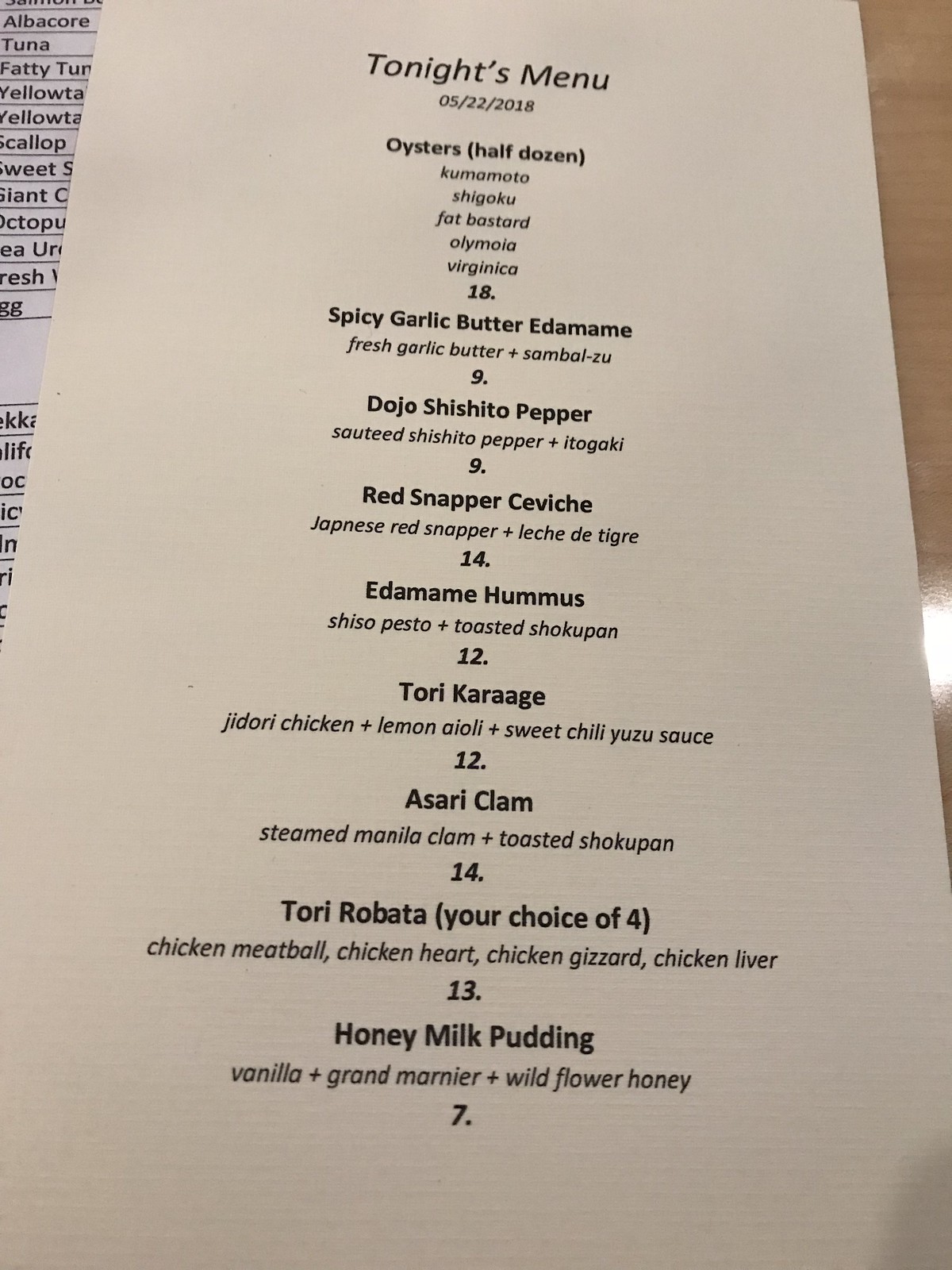This photograph captures a close-up view of a menu, arranged in portrait mode. In the upper left-hand corner to the left-center, the menu appears to be layered over another piece of paper, revealing just a sliver of it beneath. In this same area, a white chart lists various items, though the text is partly ambiguous. Some identifiable items include "albacore tuna," "fatty tuna," "yellowtail," "scallop," "sweet shrimp," "giant clam," "octopus," "uni," and “fresh egg,” although some text is partly obscured and difficult to read.

Moving to the upper right-hand corner to the right side, the menu lies on a shiny, light brown surface, likely a table, with visible lighting reflecting off its polished finish. The menu itself is printed on heavy-weight, dark cream paper.

At the very top of the menu, the heading reads "Tonight's Menu 05.22.2018," followed by a list of dishes and their prices:

1. **Oysters Half Dozen** 
    - Varieties: Kumamoto, Shigoku, Fat Bastard, Alimoya, Virginica - **$18**
2. **Spicy Garlic Butter Edamame**
    - Ingredients: Fresh garlic butter, sambal - **$9**
3. **Dojo Shishito Pepper**
    - Ingredients: Sautéed shishito pepper, ito gaki - **$9**
4. **Red Snapper Ceviche**
    - Description: Japanese (misspelled as 'Japnese') red snapper, leche de tigre - **$14**
5. **Edamame Hummus**
    - Ingredients: Shiso pesto, toasted shokupan - **$12**
6. **Tori Karaage**
    - Description: Jidori chicken, lemon aioli (incorrectly described as Italian for oil and garlic), sweet chili yuzu sauce - **$12**
7. **Asari Clam**
    - Description: Steamed Manila clam, toasted shokupan - **$14**
8. **Tori Robata**
    - Choice of: Chicken meatball, chicken heart, chicken gizzard, chicken liver - **$13**
9. **Honey Milk Pudding**
    - Ingredients: Vanilla, Grand Marnier, wildflower honey - **$7**

Each dish is accompanied by a price, indicating the cost in dollars, commonly denoted as 9, 14, 12, etc., validating the assumption about the pricing format.